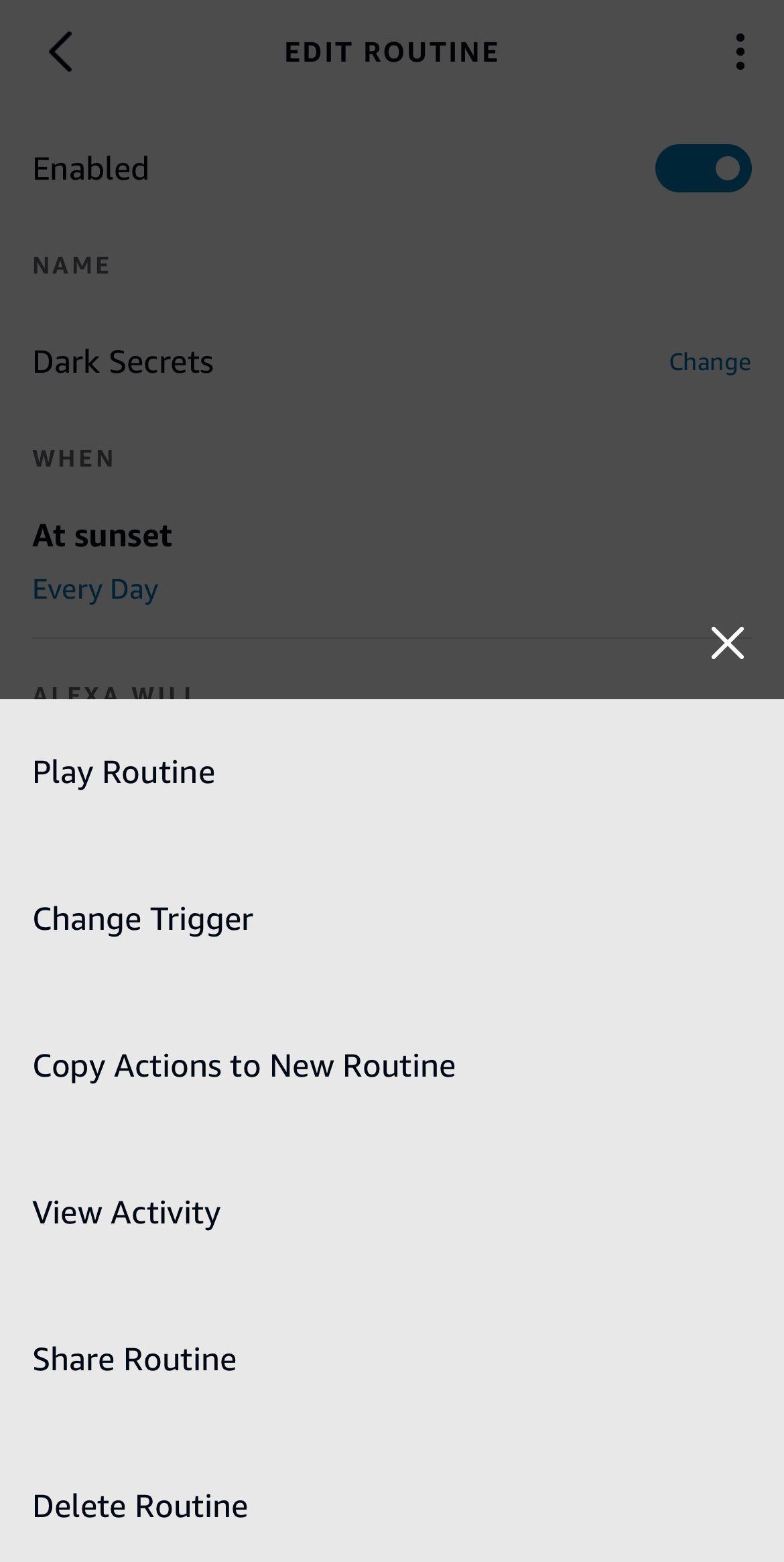In this mobile phone screenshot, the upper half of the screen features a dark gray rectangle with a white "X" located in its bottom right corner. Below this, the screen transitions to a light gray background that extends to the bottom. 

The interface presents several options in black text, each separated by noticeable spacing:
- "Play Routine"
- "Change Trigger"
- "Copy Actions to New Routine"
- "View Activity"
- "Share Routine"
- "Delete Routine"

At the top left within the gray box, there is a dark gray left-pointing arrow. Centrally positioned at the top in dark gray capital letters is the text "EDIT ROUTINE." The top right corner shows a vertical ellipsis (three dots stacked vertically). 

Directly below this header, there is an indicator showing the status of the routine. It includes black text that reads "Enabled" with a blue toggle slider set to the "on" position (white circle to the right). 

Further down, the label "NAME" appears in gray uppercase letters, followed by the routine name "Dark Secrets" in black text. To the right of this is a blue text link that says "Change."

Continuing downwards, the word "WHEN" is displayed in gray capital letters, with "at sunset" presented in black text beneath it. This is followed by "everyday" in blue text. 

A gray horizontal line separates these sections.